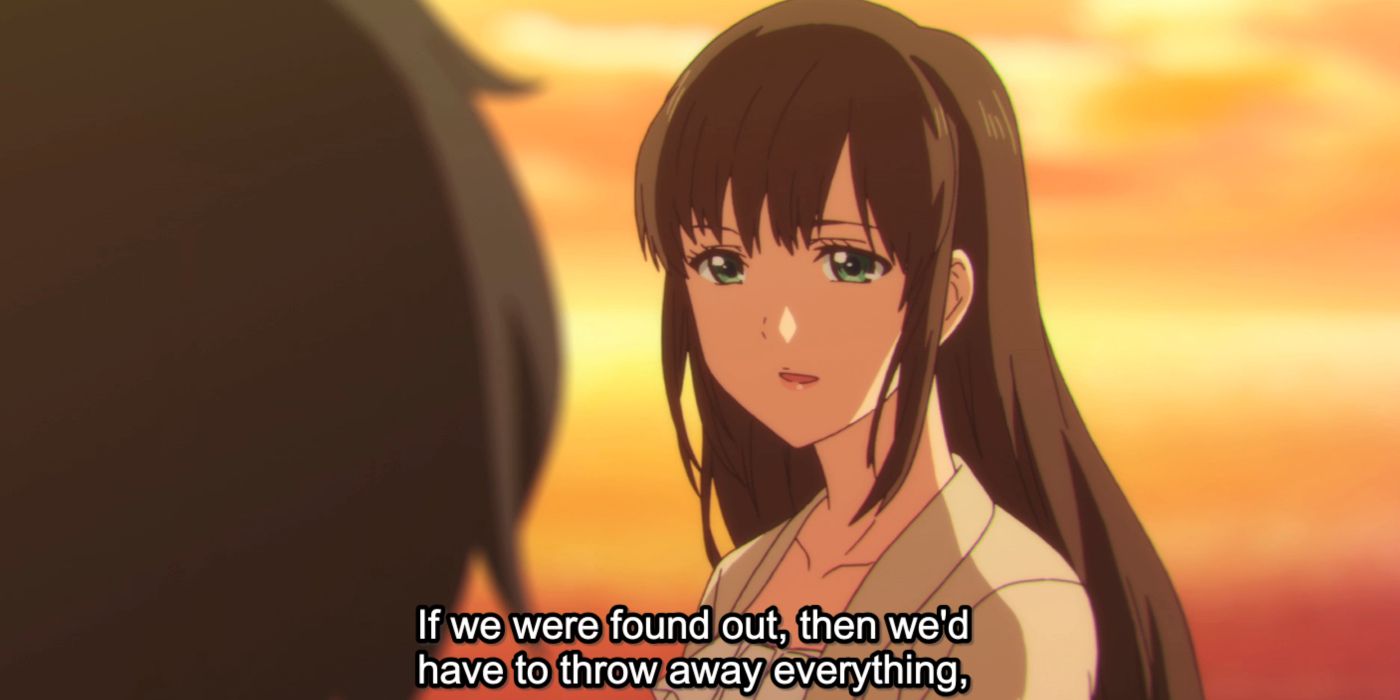The image is a detailed scene from a Japanese anime, capturing an emotionally intense conversation between two characters. At the center of the frame is a young girl with long brown hair and striking green eyes. Her hair, styled with long bangs, flows down her back, complementing her pale peach skin and pointy chin. She wears a tan-colored top, and her small mouth and ear are subtly visible. The girl is the focal point, sharply in focus against a blurred background, suggesting a deep moment of reflection or conversation.

The background is a picturesque sunset, with streaks of orange, yellow, and red painting the sky in muted tones. This creates a warm yet somber atmosphere, enhancing the emotional weight of the scene. The subtitle at the bottom of the image reads, "If we were found out, then we'd have to throw away everything," hinting at a significant and secretive context within the narrative.

In the foreground, slightly blurred, is another character with short brunette hair, suggesting a male figure due to the hair length and style. The perspective only allows the back of this person's head to be seen, emphasizing the girl's expressive, deep green eyes as she gazes towards them, adding depth to the depicted interaction.